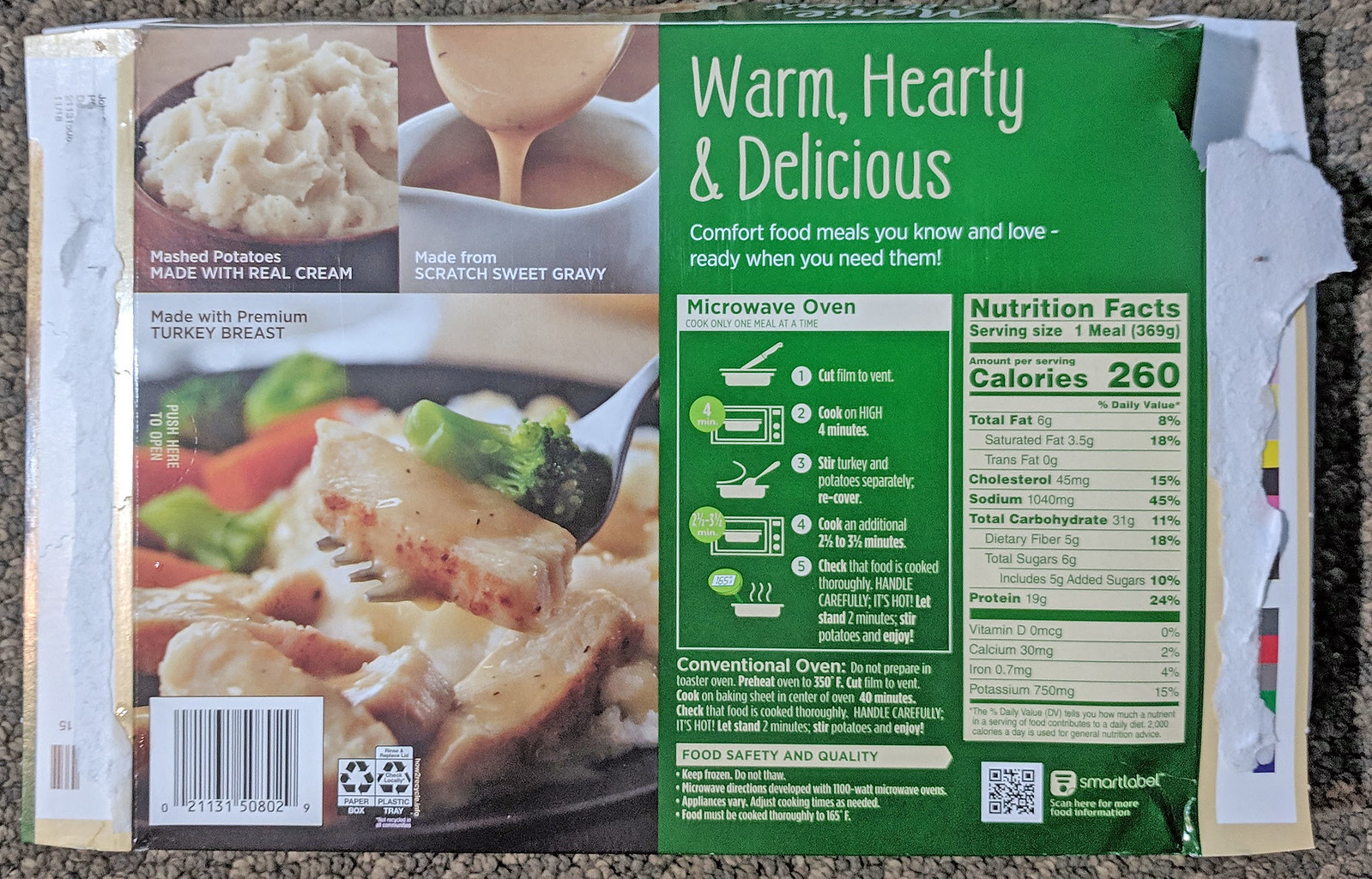This detailed caption could be used for the photo of the back of a carton of frozen dinner:

---
On the left side of the back of the carton, a series of high-quality images showcase the components of the meal, emphasizing its appeal. At the top left, a photograph of creamy mashed potatoes highlights the text, "Mashed Potatoes made with Real Cream." Directly below, an image captures rich brown gravy being poured from a spoon into a pristine white container, accompanied by the text, "Made from Scratch Sweet Gravy." Further down, a photo depicts slices of premium turkey breast arranged on a plate, with one slice held up by a fork accompanied by a piece of green broccoli, demonstrating the quality conveyed by the text, "Made with Premium Turkey Breast." These descriptive images on the left side of the box vividly illustrate the enticing meal elements. On the right side, the nutritional facts and cooking instructions are clearly displayed, providing essential information for the consumer.
---